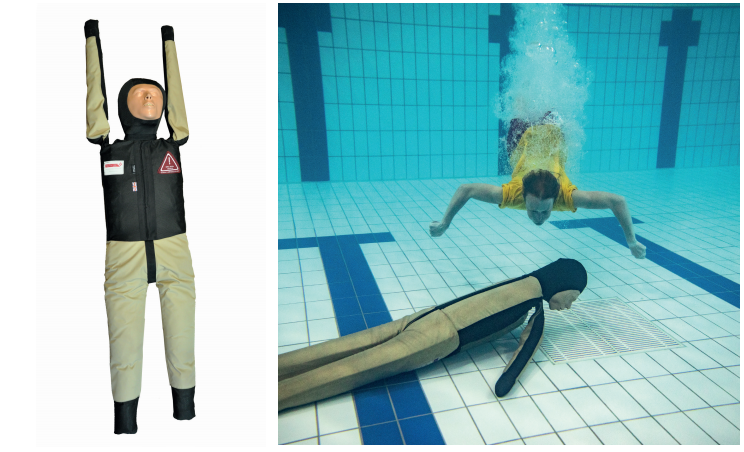The image is a composite of two full-color photographs arranged in a square format. The smaller, vertically rectangular photo on the left shows a rescue dummy dressed in a black hooded top with tan sleeves and pant legs, and small badges on the chest area. The dummy, with its arms raised above its head, is lying on a concrete surface.

The larger, square photograph on the right captures a detailed underwater scene inside a large, brightly lit pool with white and blue tiled flooring. The rescue dummy is seen face-down on the pool's floor, appearing to rest near a filter. A Caucasian male, wearing a white t-shirt and blue shorts, has just dove into the water, creating a cloud of bubbles behind him. He appears to be in the act of rescuing the dummy, suggesting this is a training exercise. The water is clear, and the scene is well-lit, allowing for vivid visibility.